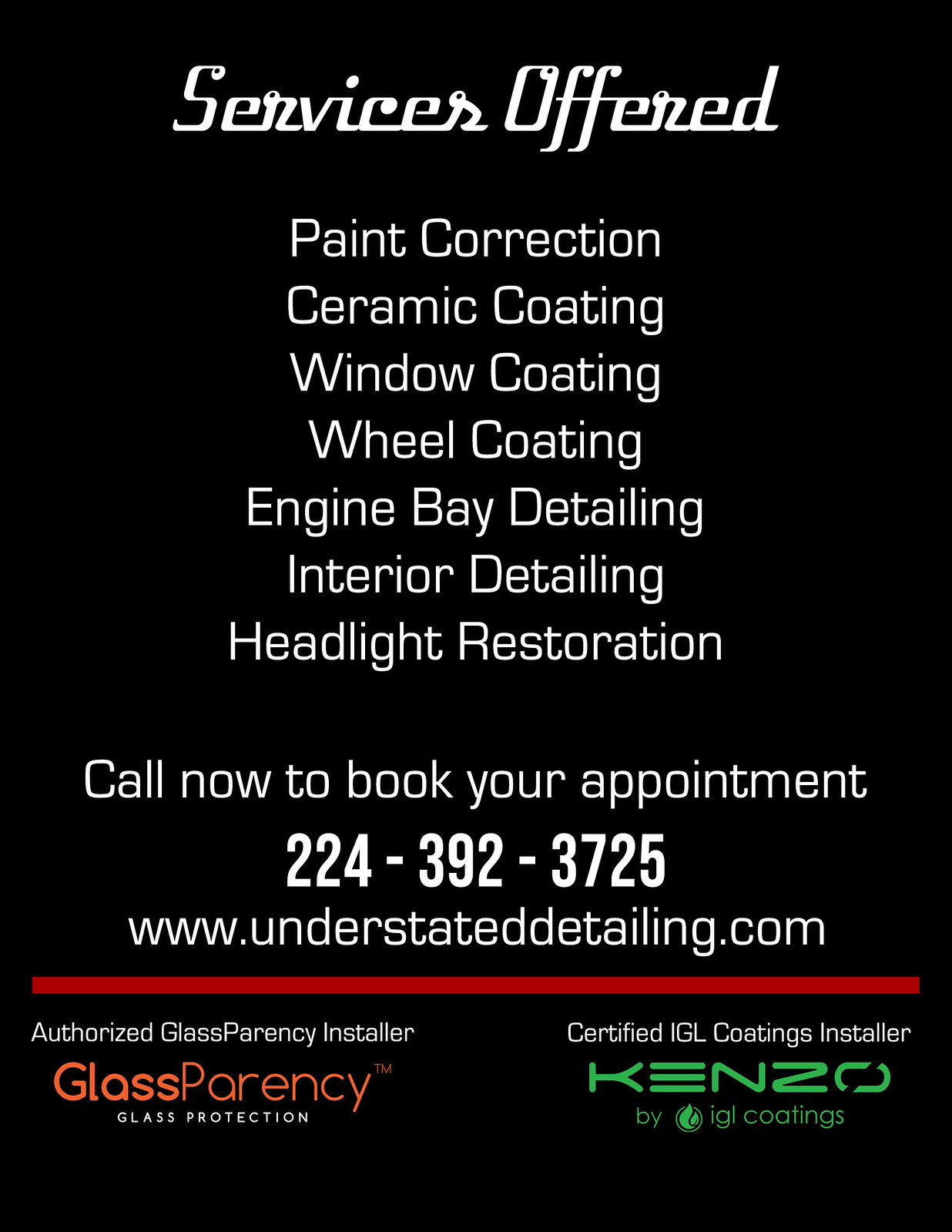The advertisement page features a black background with "Services Offered" prominently displayed at the top in white letters. Below this header, a detailed list of services is provided: Paint Correction, Ceramic Coating, Window Coating, Wheel Coating, Engine Bay Detailing, Interior Detailing, and Headlight Restoration—all written in white text. Beneath the service list, there is an invitation to "Call now to book your appointment" followed by the phone number 224-392-3725, and the website, www.understateddetailing.com. A red horizontal divider line separates these details from additional content below. On the bottom left side, "GlassParency" is highlighted in vibrant red letters, accompanied by the text "Glass Protection" and "Authorized GlassParency Installer" beneath it. On the bottom right, it states "Certified IGL Coatings Installer," with "Kenzo by IGL Coatings" written in green letters.